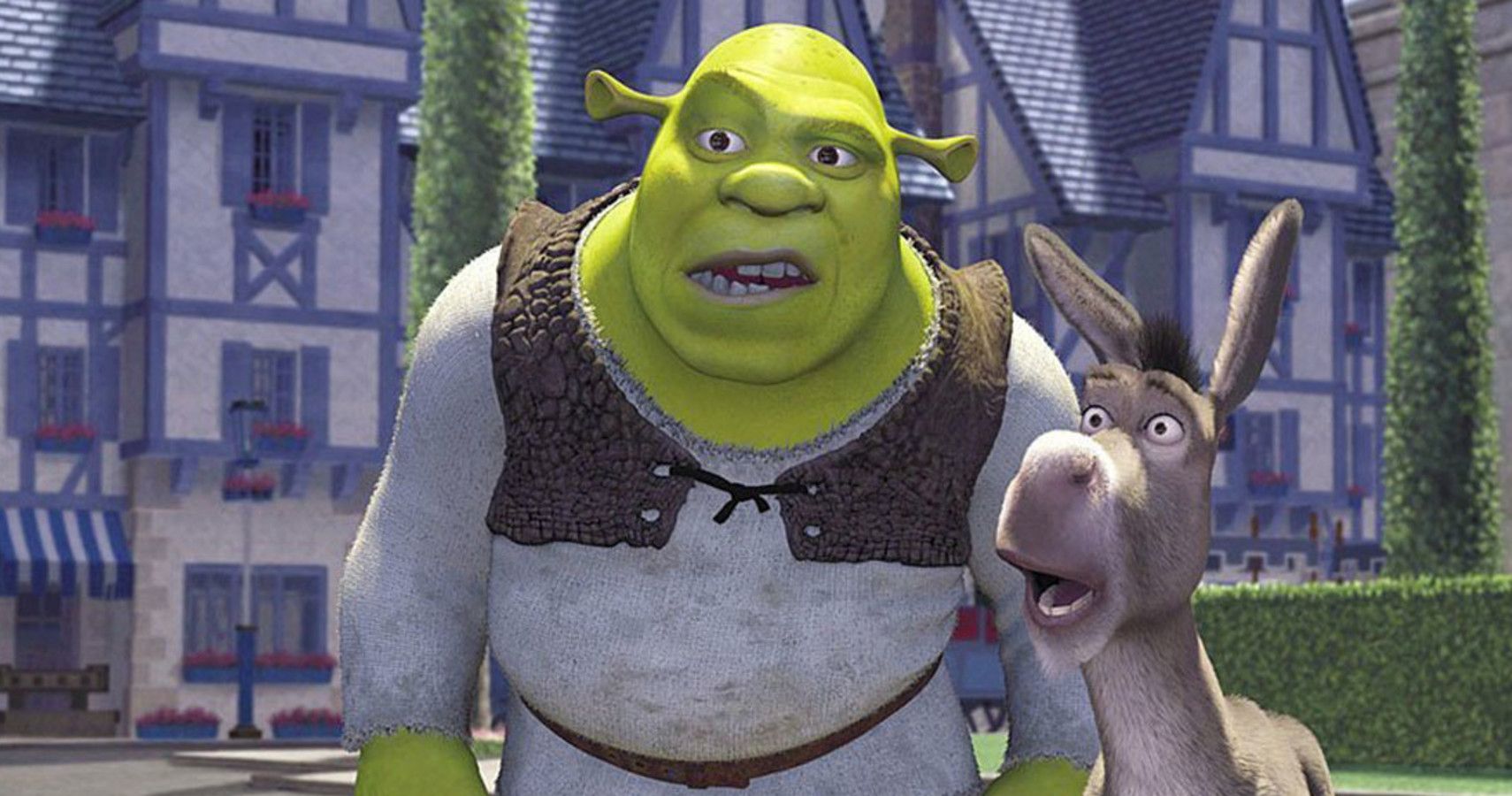This detailed still from the 3D animation movie "Shrek" prominently features the main character, Shrek, and his friend Donkey. They stand in an outdoor setting, both showing expressions of surprise and confusion. Shrek, a bright green ogre with human-like eyes, mouth, and nose, is depicted from the torso up. He sports small, cylindrical ears on either side of his bald head, wears a white long-sleeve shirt under a brown vest, and has a brown belt around his waist. To Shrek's right is Donkey, who exhibits a very surprised look with wide, bugging-open eyes. Donkey is mostly gray with white markings on his mouth, nose, and the front of his neck, and has a distinct black mohawk. The background features a cityscape with white houses trimmed in blue, tall trees, green shrubs, and a garden area, contributing to the animated outdoor scene.